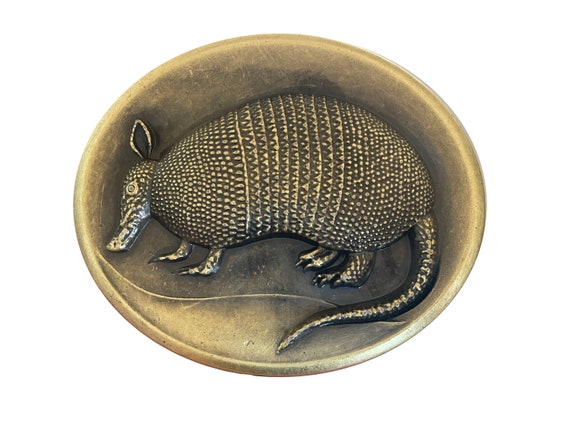This photograph features a possibly brass, oval-shaped medallion that appears to be fairly old and worn. The medallion exhibits a gradient of colors, transitioning from a shinier, golden hue along the edges to a darker, more aged appearance in the center. In the middle of the medallion, there is a detailed carving of an armadillo facing right. The armadillo showcases a textured, armored shell with distinct bumps, a long tail that curves down and tucks beneath towards the bottom center of the medallion, and short, claw-like feet. The carving also includes a prominent single eye and tall ears, though only one ear is fully visible, with the other being a faint outline. The background of the image is plain white, emphasizing the intricate details and wear of the medallion.